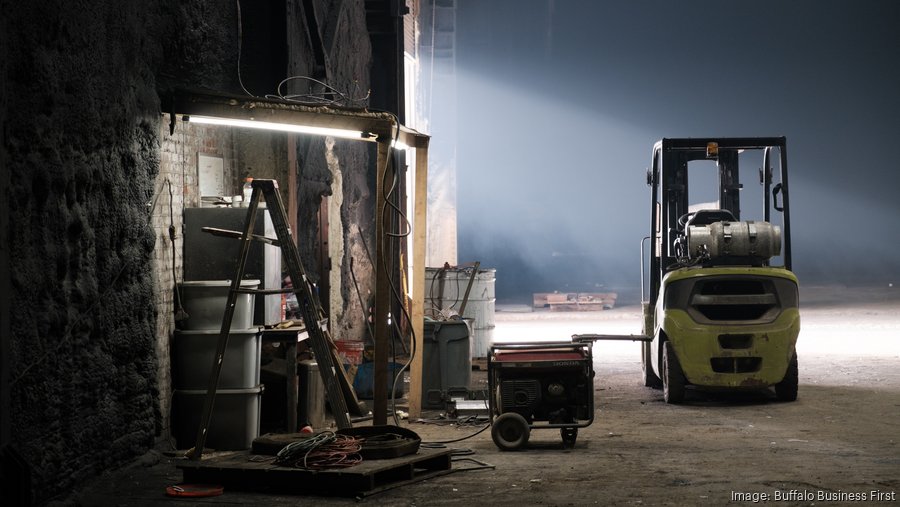This photograph captures the interior of what seems to be an abandoned factory. The scene is dominated by a neon green and black forklift, the type typically used for moving pallets of products in industrial settings. The forklift stands in the middle of a spacious area with a dirt floor. The factory is dimly lit, but daylight streams in through a large bay door on the left, casting an ethereal, foggy light across the floor due to the dust particles suspended in the air.

On the left side of the image, a small shack used for storing containers is visible, surrounded by Tupperware crates and various industrial materials, including pipes and a U-shaped wooden frame emerging from the ground. This frame is outfitted with fluorescent lights to partially illuminate the otherwise dark space. Additional elements like a wooden ladder and stray wires scattered on the ground contribute to the disarray. A watermark at the bottom right corner reads "Buffalo Business First," subtly indicating the source of the photograph.